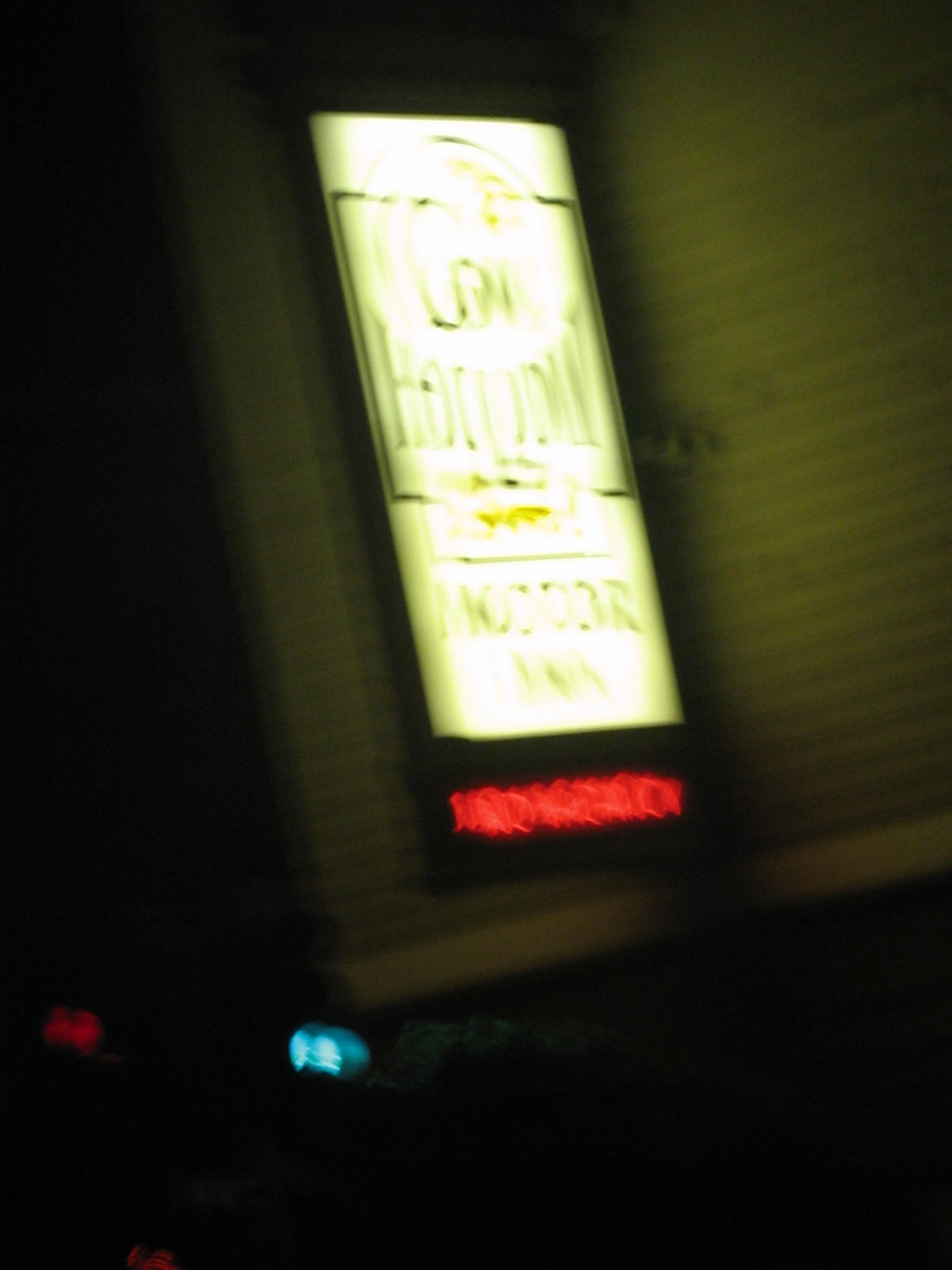The photograph, taken at night, is noticeably blurry. It captures an illuminated sign, presumably for a business, although the business name is indiscernible due to the light glare and blurriness. The main sign is white with black and possibly some gold text. Below this sign is another smaller, red illuminated sign which seems to say "No Vacancy," though its legibility is compromised by the blurriness. The background reveals white siding where the signs are mounted, and the corner of the image faintly shows red and blue lights.